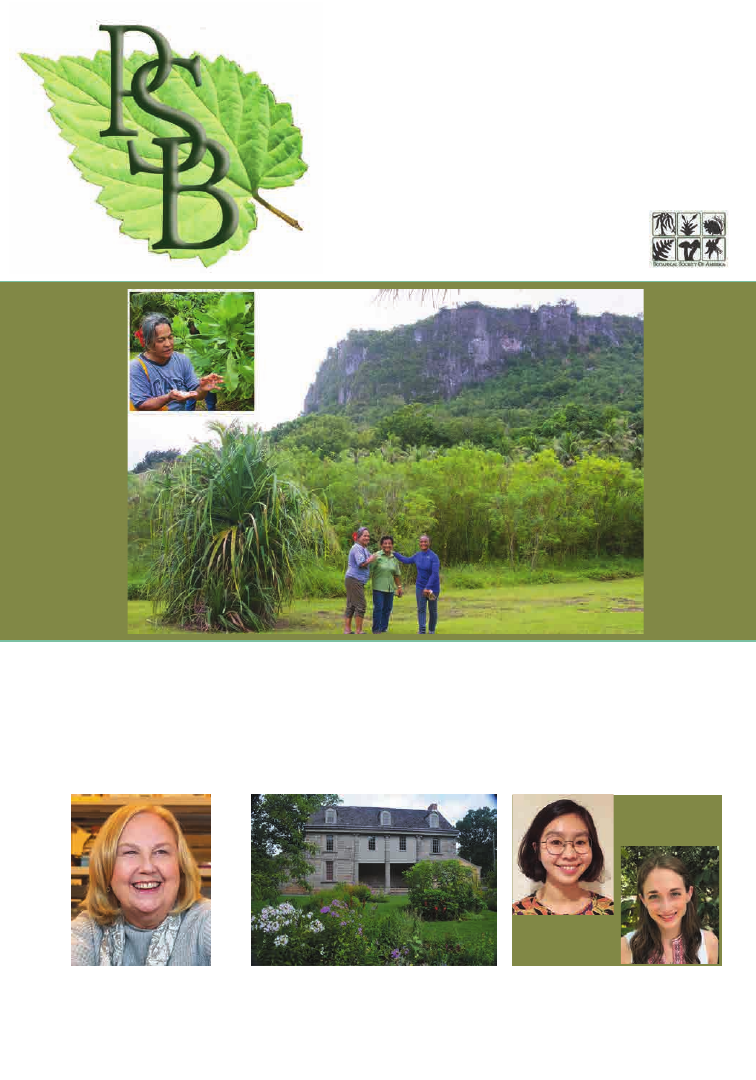This advertisement showcases a collage of images set against a white background, with the topmost section featuring a green leaf with "PSB" written in black letters over it. Below this, an olive green horizontal rectangle frames the central image, depicting three individuals standing in an open, green field with tall trees behind them. In the distant background, a large rocky cliffside, dark and purplish, rises high with a hint of possible structures at its summit.

Beneath the main image are three smaller photos arranged horizontally. From left to right, the first photo captures a light-skinned blonde woman with shoulder-length hair, dressed in a light blue-patterned scarf and a light blue-white blouse. The second photo in the center showcases an elegant European mansion set amidst a field, adorned with bushes and flowers. The third photo features two young women smiling, one with dark hair and round glasses, and the other with dark hair cascading over her shoulders, wearing a white blouse. Finally, in the upper left corner of the collage, a small vertical image shows a close-up of a woman with a flower in her hair, seemingly focused on something in her hands.